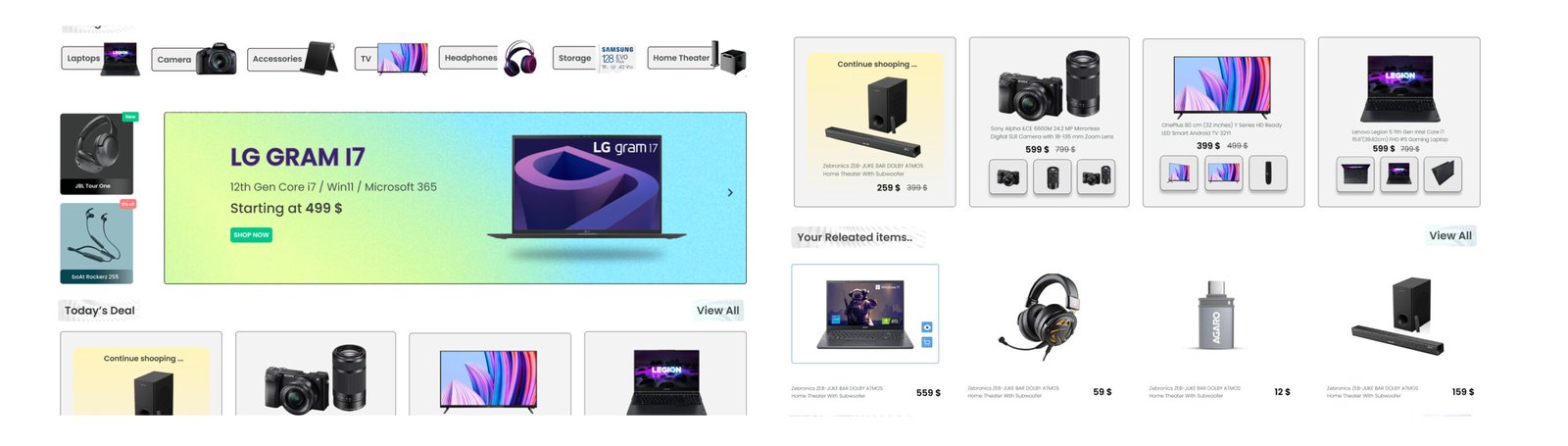Two adjacent screenshots from an electronics store website, displayed side by side against a very light background, either white or light gray. Each product listing is enclosed in a light gray box with a slightly darker gray outline or drop shadow. A range of electronic products is featured, including a camera, a big screen TV, a laptop, a headset, and a sound bar with a subwoofer.

The left screenshot prominently features a large banner ad for the LG Gram 17 laptop, extending over a significant portion of the screen. The ad boasts a gradient background of light green and light blue, with purple text announcing "LG Gram 17" and specifications such as "12th Gen Core i7," "Windows 11," and "Microsoft 365." The price starts at $499, with a "Shop Now" button included. The laptop image showcases the screen and keyboard, set against a transparent background on the gradient.

The left screenshot also includes a bit of a menu bar on its left side. The adjacent right screenshot continues with more product listings, effectively completing the cut-off portion from the left image. This layout indicates it's part of an extended view of the same online store, providing a broader display of available electronics.